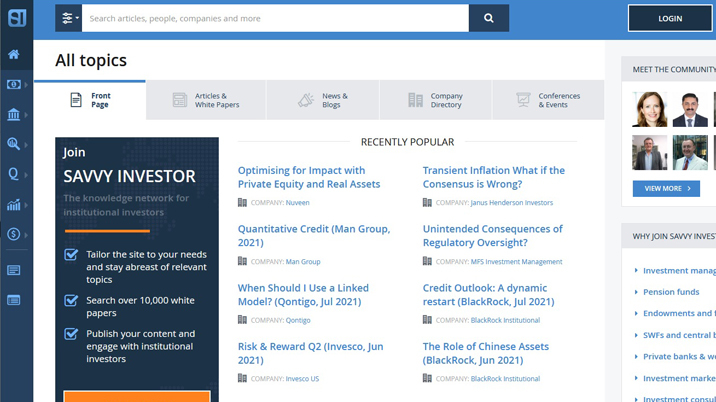The image features a predominantly white background. Across the top, a light blue banner spans the width of the layout, housing a prominent search box and a login button. Below the light blue banner, the white background displays the text "All Topics" underlined with a blue line. There is a small icon of a page labeled "Front Page" adjacent to a series of categorized blue boxes containing titles such as "Articles and White Papers," "News and Blogs," "Company Directory," and "Conferences and Events."

On the left side, a dark blue vertical box runs down the length of the image. Within this dark blue box are multiple smaller icons and graphics: a small blue box followed by a house icon, another smaller box with a circle inside it, another house, a magnifying glass, the letter 'E', another house, a circle featuring a dollar sign, and two paper icons representing different document types.

At the top of the dark blue section, an embedded bold dark blue box states "Join Savvy Investigator" underscored with an orange line. Below this, text explains the benefits of customizing the site, staying informed on relevant topics, searching through 10,000 white papers, publishing content, and engaging with institutional investors. This portion also features checkmark icons highlighting each benefit, all underlined by another orange line.

Centrally located in the image, a section titled "Recently Popular" lists several items that are currently trending. On the far right, the "Meet the Community" segment displays four thumbnail snapshots of community members and a blue "View More" button, adjacent to "Why Join Savvy Investments," which lists various advantages of joining the platform.